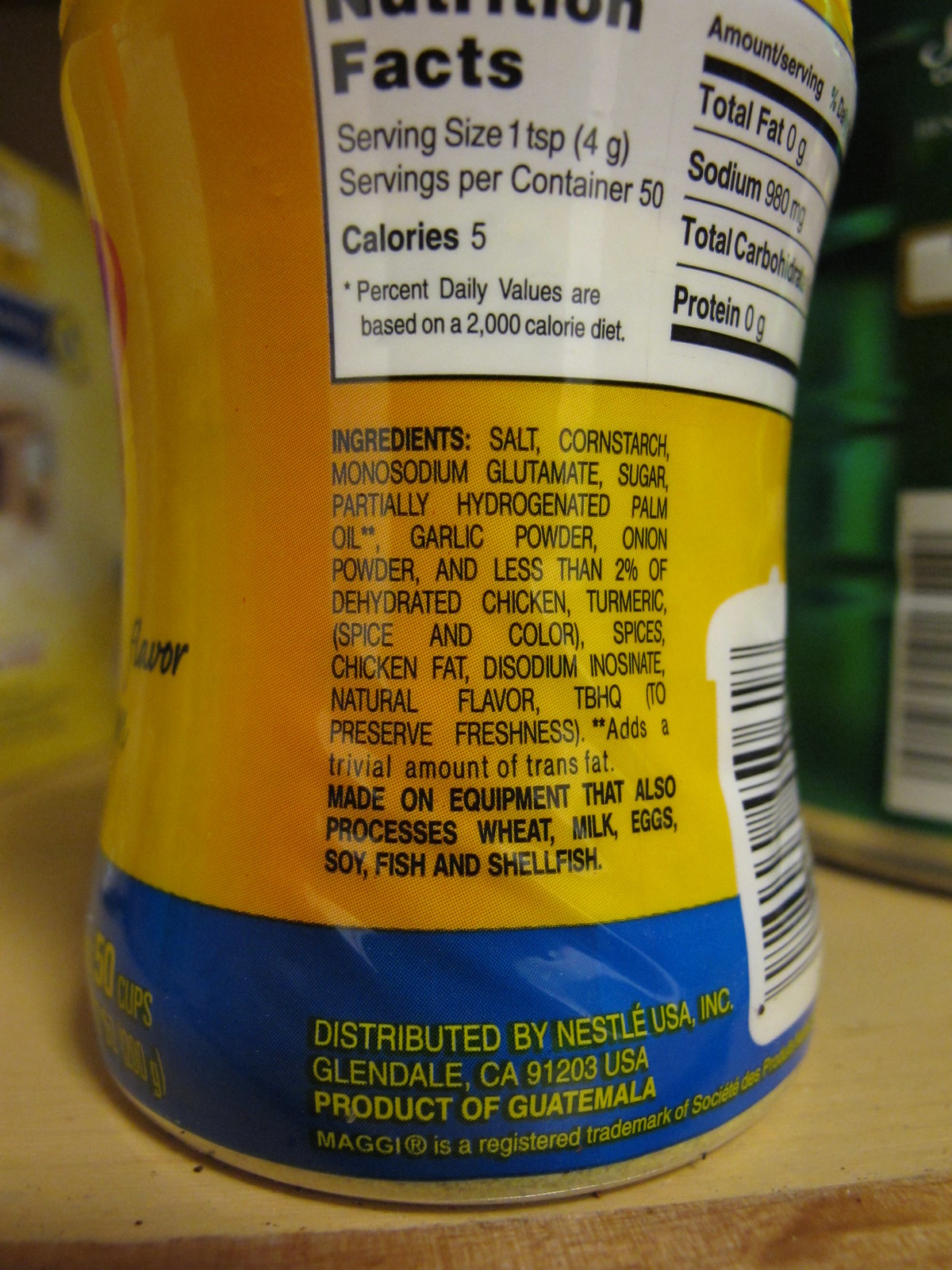This is a color photograph depicting the back of a food item bottle, showcasing its nutrition facts and ingredient list. The label, primarily orange-yellow with a darker blue section at the bottom featuring yellow lettering, is slightly curved, revealing the nutritional information on a white rectangular background. The label details a serving size of 1 teaspoon (4 grams), with 50 servings per container, and 5 calories per serving, noting that the percent daily values are based on a 2,000 calorie diet. The ingredient list below reads: salt, cornstarch, MSG, sugar, partially hydrogenated palm oil, garlic powder, onion powder, less than 2% of dehydrated chicken, turmeric (for spice and color), additional spices, chicken fat, disodium inosinate, natural flavor, and TBHQ to preserve freshness, with a note that the palm oil adds a trivial amount of trans fats. The bottle is a product of Guatemala and is distributed by Nestle USA Inc., Glendale, CA, 91203, USA. The photo also includes a visible barcode on the right side, and the bottle is placed on a brownish counter, with blurred food containers in the background.